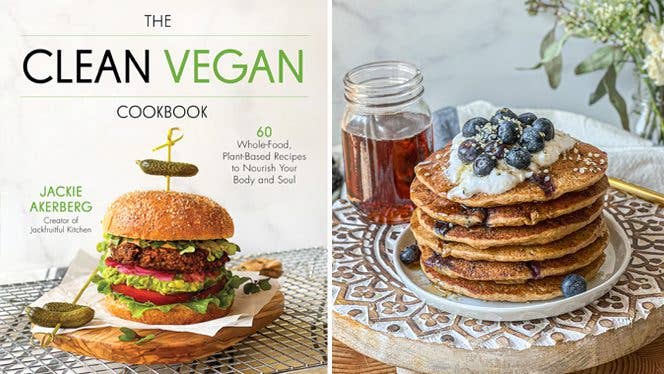The image shows two pictures side by side. The left picture is the cover of "The Clean Vegan Cookbook" by Jackie Akerberg, the creator of Jack Fruitful Kitchen. The title features black text, except for the word "Vegan" which is in green. Central to the cover is a high-stacked vegan hamburger, comprising a red-brown bun, layers of smashed avocado, tomato, lettuce, and a patty. There is a small pickle or cornichon skewered with a plastic sword sticking through the top bun, and two more cornichons are laying on the left side of the burger, which sits on a wooden cutting board. Below the title, the cover also highlights, "60 whole food plant-based recipes to nourish your body and soul."

The right picture showcases a stack of browned blueberry pancakes topped with fresh blueberries and whipped cream. These pancakes are arranged neatly on a small white plate with a lip, and to the side, there is a jar of what appears to be maple syrup. The scene is completed with a sunburst-patterned ceramic piece beneath the plate and a vase of flowers in the background, adding a homely touch to the setup.